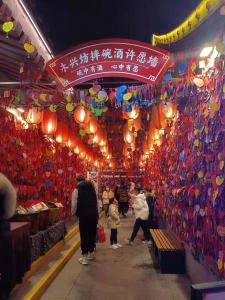This vibrant photograph, possibly taken in Chinatown or China, captures a lively, narrow corridor illuminated by rows of glowing Chinese lanterns stretching from the foreground to the background. The scene is filled with colorful decorations in shades of red, yellow, blue, and purple adorning both sides of the walkway. These vibrant displays include intricate ribbons or possibly paper decorations hanging along the corridor, enhancing the festive atmosphere. At the top, a bright red semicircular banner with Chinese characters is prominently displayed, suggesting the location or the nature of the celebration. The image, taken at night, reveals a bustling scene with people, including children and a family, exploring the area. On the left side, a man appears to be examining something, possibly at a food stall, while the right side is solely decorated. The overall setting, with benches for resting and the illuminated lanterns, evokes a sense of an open-air market or shopping area, capturing a modern snapshot of a joyous celebration.